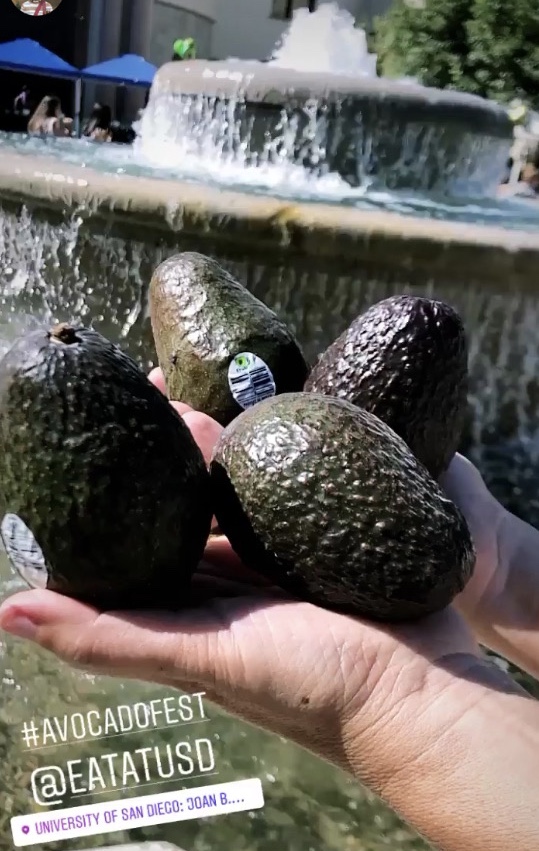In this bright outdoor photograph taken in sunlight, a pair of hands enters the frame from the lower right, palms up, holding four large avocados. The avocados are a mix of green and dark green, almost purple hues, with one featuring an unreadable white oval label. In the background, there is a multi-tiered, circular cement fountain with water spirting and cascading down its levels. Further back, vibrant blue umbrella-covered tables are visible, with people seated at them. Overlay text at the bottom left of the image reads "#AvocadoFest" and "@eat at USD." Below this, a white rectangle with purple text states "University of San Diego Joan B." The setting suggests a festive environment, possibly a campus event.